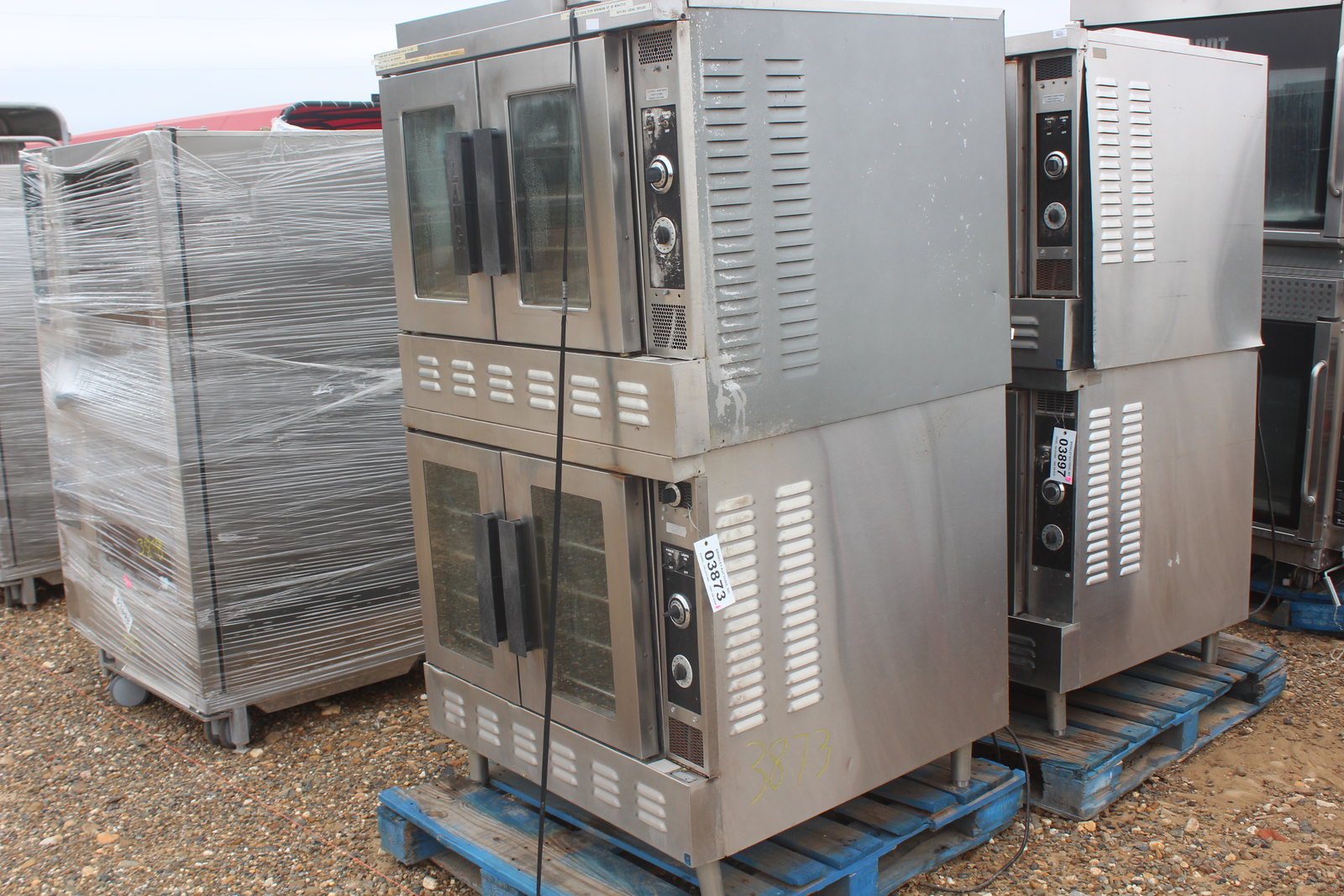In the image, we see an outdoor storage area where large industrial appliances are being housed. Dominating the foreground are four massive ovens, typically found in restaurant kitchens or food preparation areas. These appliances, constructed of stainless or silver metal, appear somewhat aged and show signs of wear. Each oven features two black-handled doors with glass windows, allowing a view inside, and has an open grill area at the bottom along with side grills positioned near the right-hand knobs.

The ovens are stacked on blue pallets for ease of movement, with some wrapped in protective film while the ones in focus remain unwrapped. In the background, additional appliances are visible, although their details are less discernible due to the angle and possible obstruction by the foreground ovens. Each unit carries a tag with numbers, suggesting they are part of an organized inventory. The overall scene suggests a warehouse-like environment dedicated to storing or possibly refurbishing these large kitchen appliances.